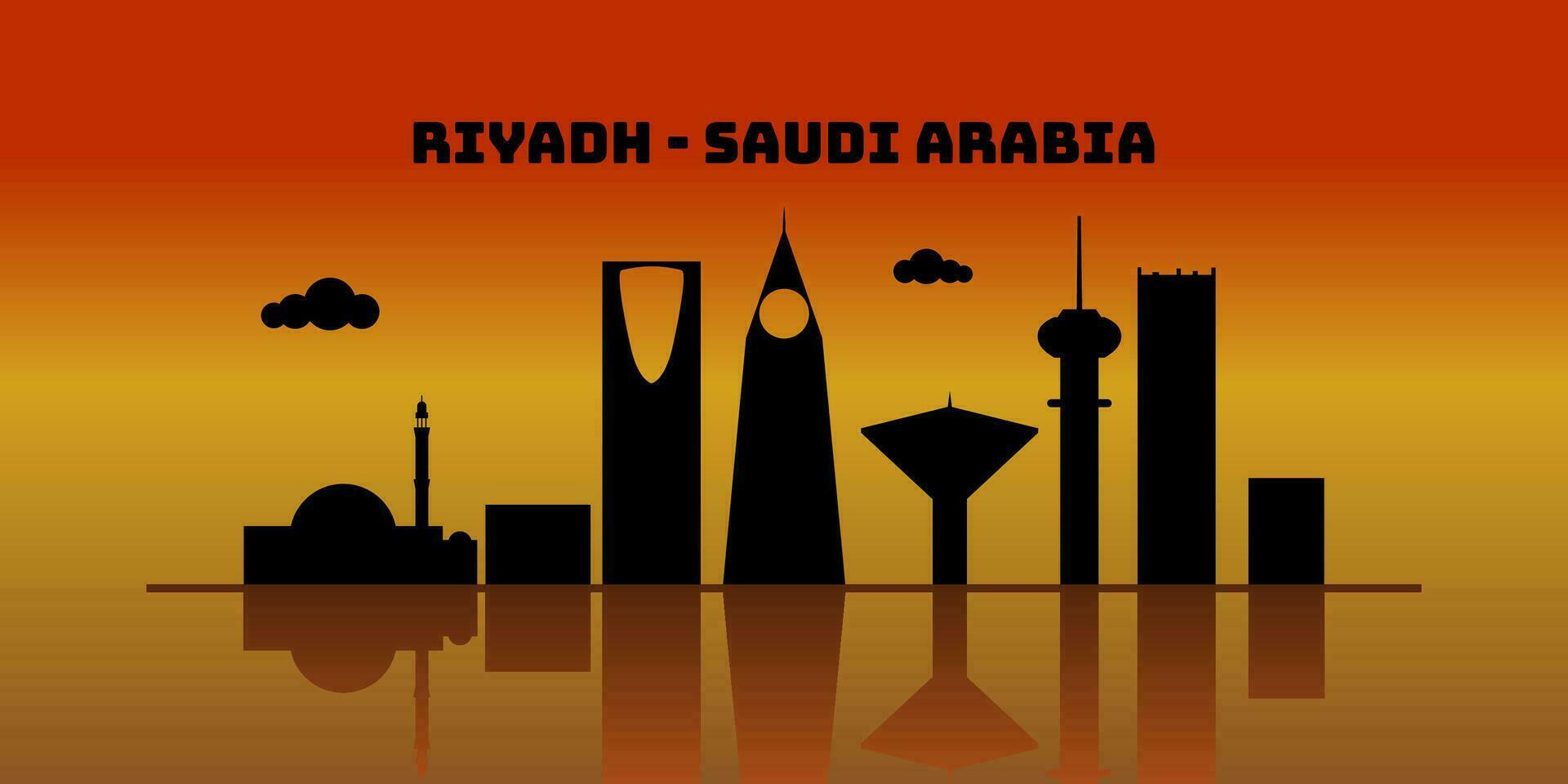The poster image, depicting the city of Riyadh in Saudi Arabia, serves as an advertisement and features a striking artistic design. Dominating the top of the image is the text "Riyadh - Saudi Arabia" in large, bold, colorful fonts. The scene is set against a warm, vivid background of oranges, reds, and yellows, suggesting the vibrant hues of a setting sun. The skyline showcases an array of buildings, blending both modern and traditional architecture, rendered in stark black silhouettes. These include renowned structures such as a mosque, a mix of square and rectangular skyscrapers, a tower with a circular top, a building resembling the Seattle Space Needle, and a structure akin to the Empire State Building.

Each building casts a reflection below, suggesting the presence of a water body. Black, shadowy puffs of clouds hover around the buildings, enhancing the dramatic aura of the scene. The juxtaposition of the bright, fiery sky and the dark, reflective buildings creates a captivating visual contrast, making the image both striking and memorable.